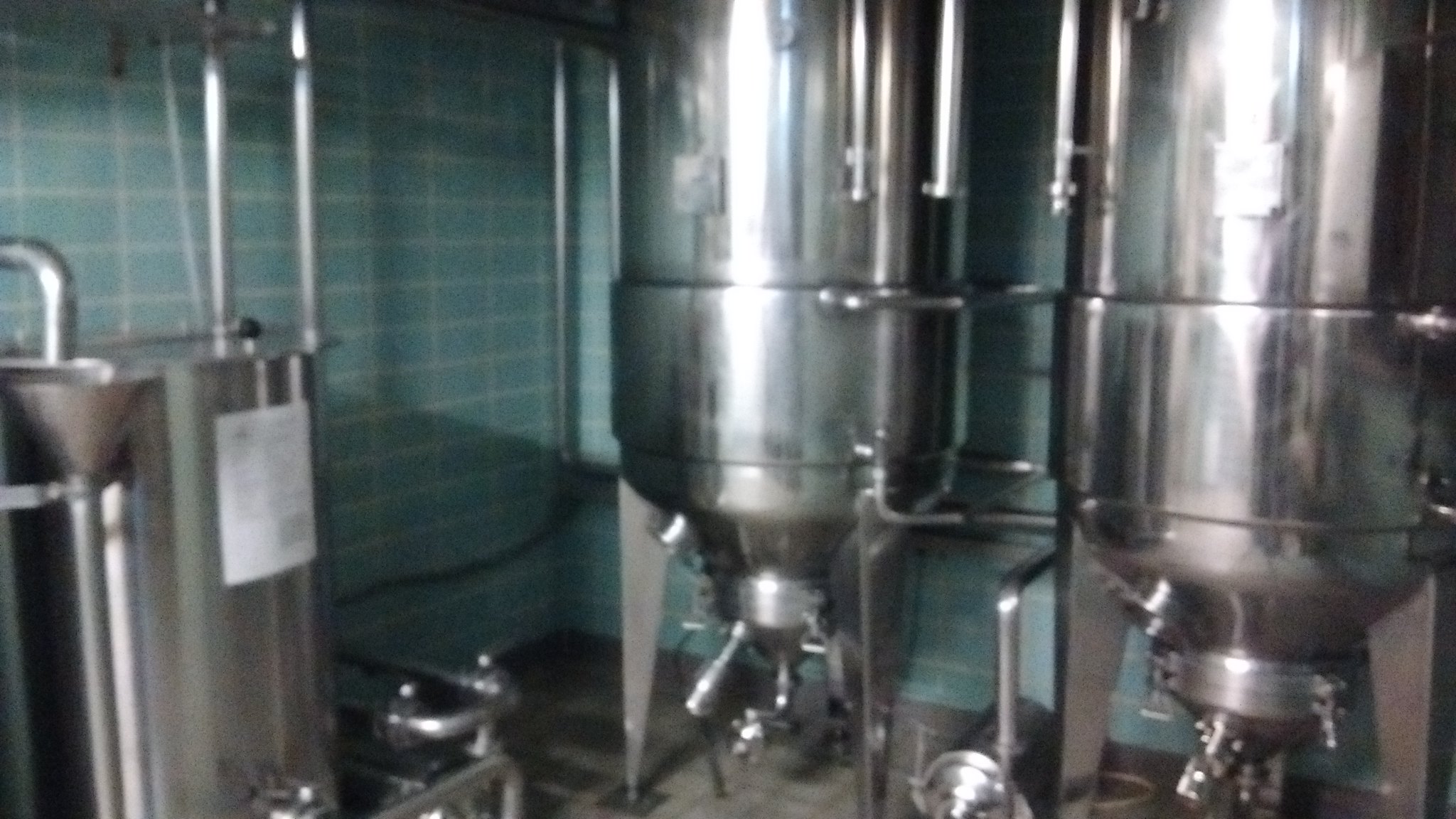The image depicts a room with light blue or teal walls tiled in small rectangular patterns, separated by white grout lines. The primary focus is on two large, silver metal cylindrical vats, commonly used in the production of alcohol. These vats are suspended from the ceiling and taper towards the bottom, each featuring multiple spouts for sampling the contents. The back wall showcases a mix of blue and white tiles. Centered between the vats is a blurry, silver motor-like apparatus on the floor, possibly used for mixing or other processing purposes. To the left, a third cylinder appears to be sliced in half with a flat top, equipped with a funnel attached to a pipe on its side, suggesting a different function. Additional piping interconnects the vats, contributing to the industrial atmosphere of the room with its gray tiled floor.